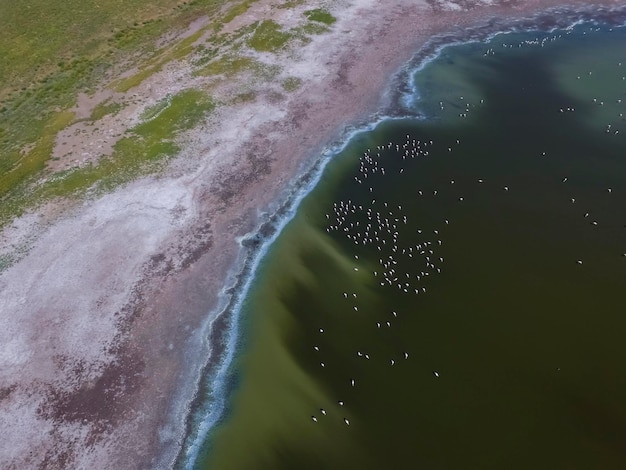This photorealistic aerial image captures a detailed view of a shoreline meeting a body of water. The beach transitions from darker brown sand to lighter brown and then to light tan as it approaches the left side of the image, where patches of green grass become more prominent. The grassy areas are interwoven with sand and some scrub brush, especially thick in the upper left corner. The water on the right is a dark green with variations of lighter green, and it appears to be covered in green algae. Scattered throughout the water and along the shoreline, there are numerous white specks, likely waterfowl such as ducks or geese. The edge of the water has slight wave breakings, adding texture to the scene. This overhead perspective suggests a viewpoint from an airplane, highlighting the varied textures and colors of the landscape below.